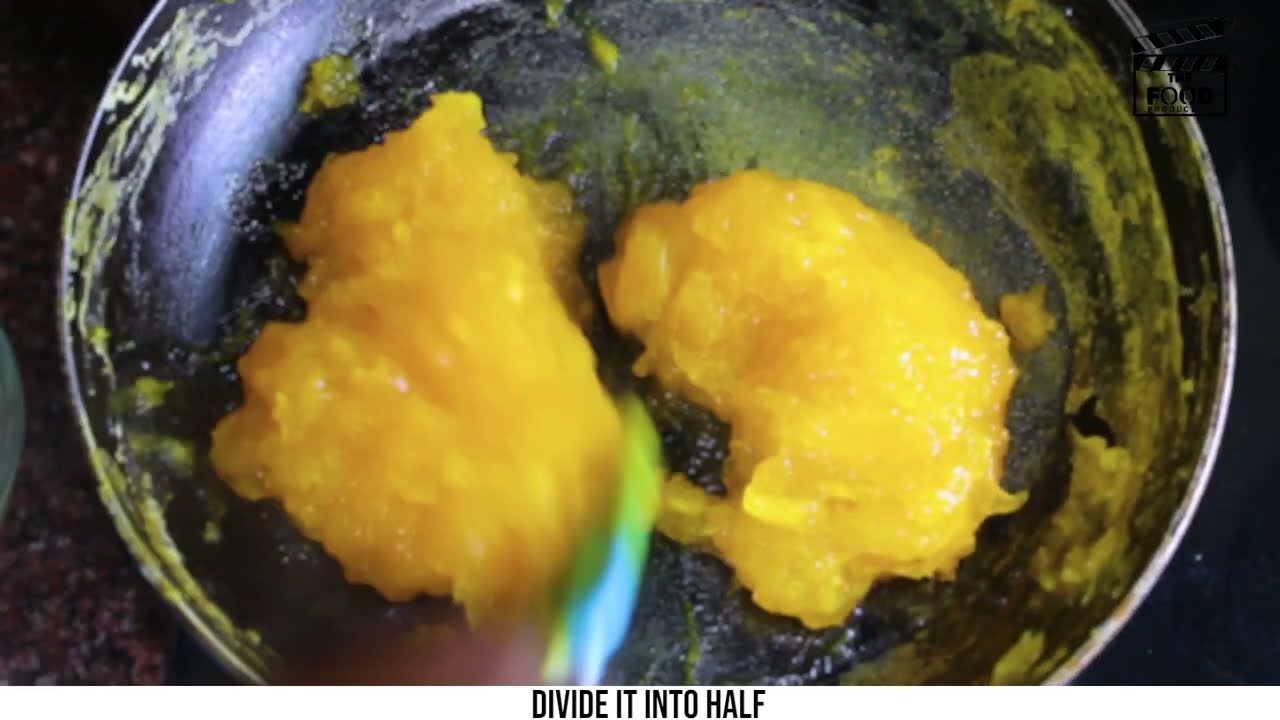In the image, we have a close-up, top-down view of a dark blue bowl that appears to be mixing a yellow substance. This yellow material has a gooey, solid consistency, resembling either mashed yellow fruit or scrambled eggs. It is divided into two uneven halves—a left portion that is pear-shaped and a right one that looks slightly rotated. A blue plastic spatula with a green tip is prominently placed in the middle, appearing slightly blurred as if in motion. The interior of the bowl is stained with the yellow substance, indicating it is sticky. Below the spatula, there is black capital text that reads "DIVIDED INTO HALF." Additionally, there's some light shining from the left side, possibly from a nearby window, and in the upper right corner, partially visible, is an icon resembling a clapperboard used in filmmaking, labeled with unreadable text. The entire scene suggests some cooking activity involving eggs or a similar yellow food, and the chaotic state of the bowl implies vigorous mixing or scrambling.